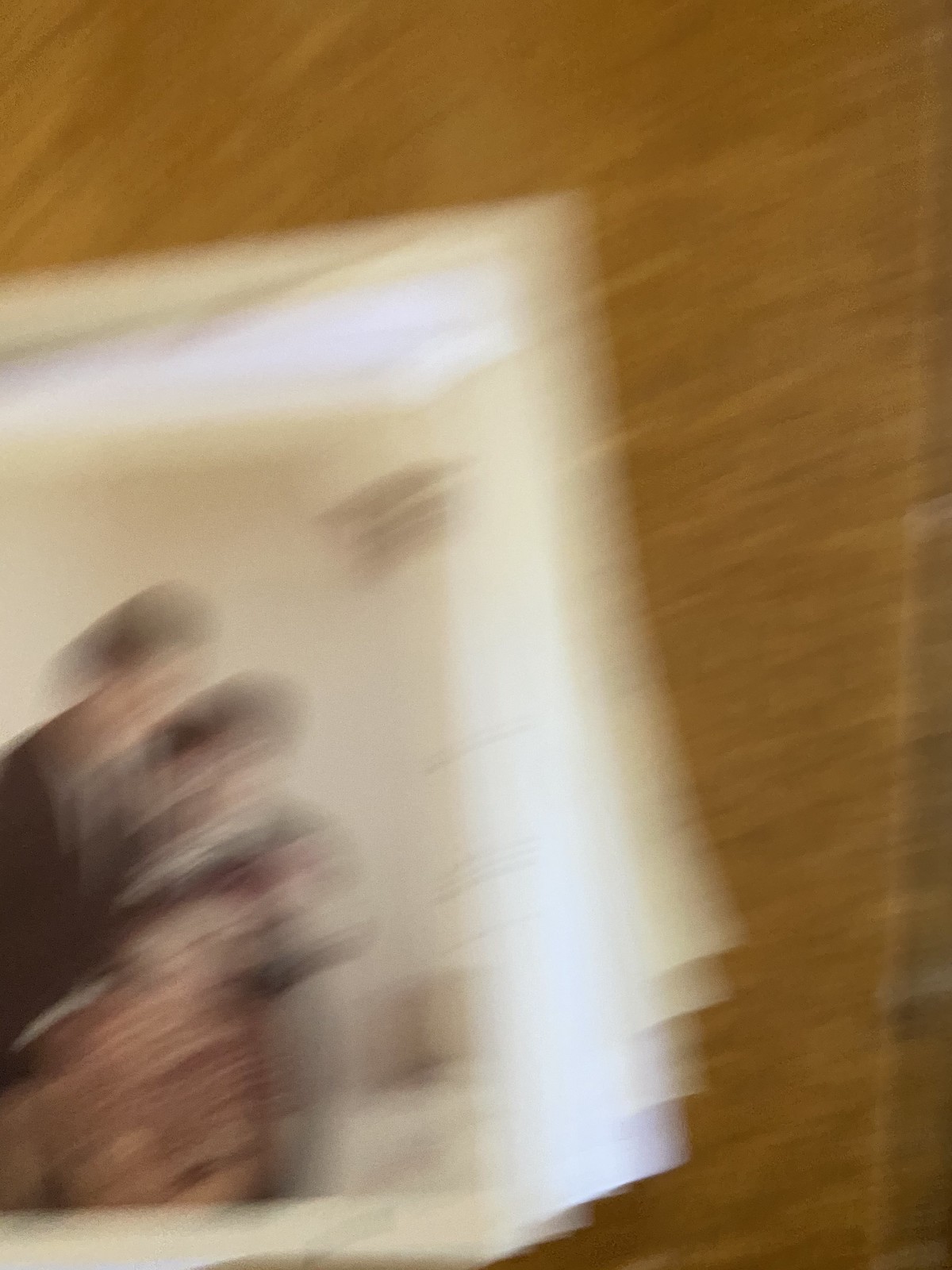The image depicts a blurry scene of a brown surface that might be wood, marked with a grainy, unclear texture. Scattered across this surface are several paper-like items that resemble photographs. Prominently, in the bottom left corner, is a particularly blurry rectangular image that seems to show a group of people—likely a family consisting of two adults and a child, or possibly another smaller child. The individual on the top left appears to be wearing a suit, while the figure to the right is dressed in gray, and there is a hint of an orangish fabric below. The individuals are lit from a bright light source on the right side, potentially a window. Above this family image, there are stacks of paper ranging in color from weathered, tea-stain hues at the top to whiter and then ivory tones beneath. The amalgamation of these details creates a sense of a textured and cluttered scene, rich in visual elements despite the overall blurriness.